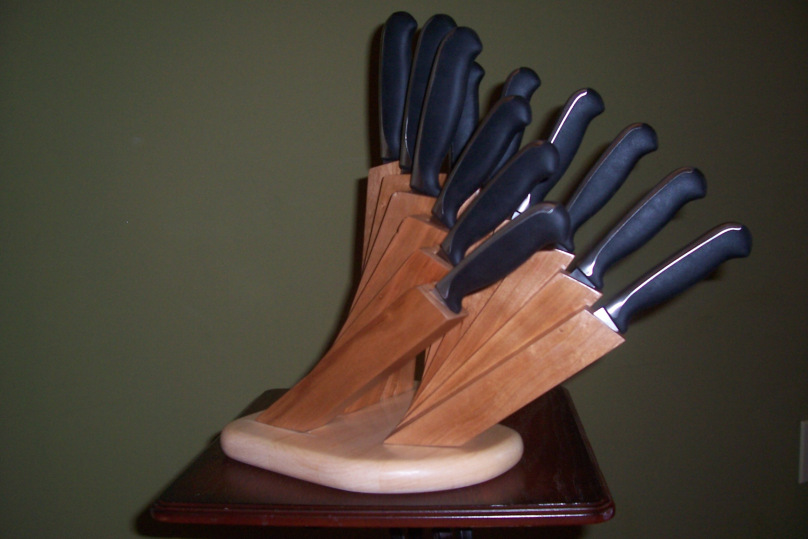This image features a striking and artistic knife holder, set against an olive-shaded, khaki green wall. The holder is stationed on a small, square table made of dark cherry or mahogany wood, enhancing the visual contrast. The knife holder itself appears to be mounted on a heavy-weight, white porcelain or marble slab, providing stability and ensuring it doesn’t tip over despite the weight of the large, black-handled knives it supports.

Comprised of two distinct sections, each containing five fanned-out wooden blocks, the holder accommodates a total of about 10 to 12 knives. The wood used is a reddish blonde or amber hue, adding to the aesthetic appeal. Each knife fits into its own individual pocket within these blocks, although they're connected at the base. The knives, primarily black-handled with occasional silvery stripes, display elegantly at various angles, from straight upright to distinct tilts to the right, making the arrangement visually captivating while also functional.